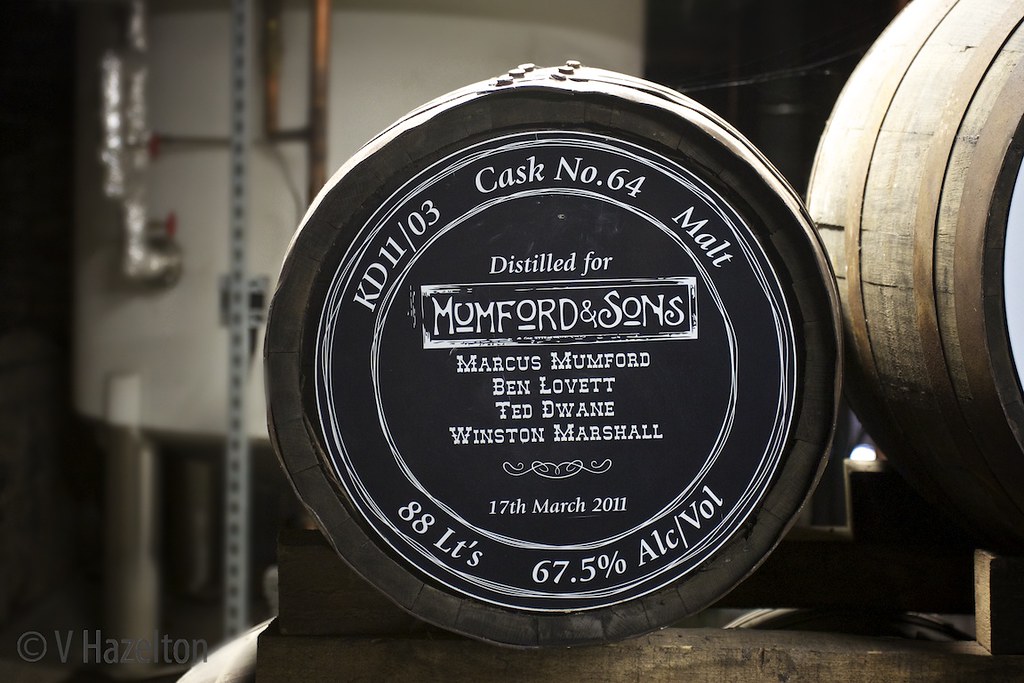In the dimly-lit distillery room, a row of oak casks is discernible under a beam of light shining from above. Central to the image, a prominent cask stands out with a detailed plaque on its front. The plaque, set against a black background with white lettering, reads: "KD11-03, Cask Number 64, Malt," and details its significance: "Distilled for Mumford & Sons, Marcus Mumford, Ben Lovett, Ted Dwayne, Winston Marshall, 17th of March, 2011." Below, it notes the cask's capacity, "88 liters," and alcohol content, "67.5% alcohol by volume." This cask is positioned at the end of a shelf, adjacent to another cask on its right. In the darkened background, a large white distillery tank with brass and metal fixtures is visible, alongside a network of pipes. The photograph, captured with a unique and modern font style by the artist V. Hazleton, focuses mainly on the labeled cask, leaving the intricate distillation machinery subtly veiled in shadow.